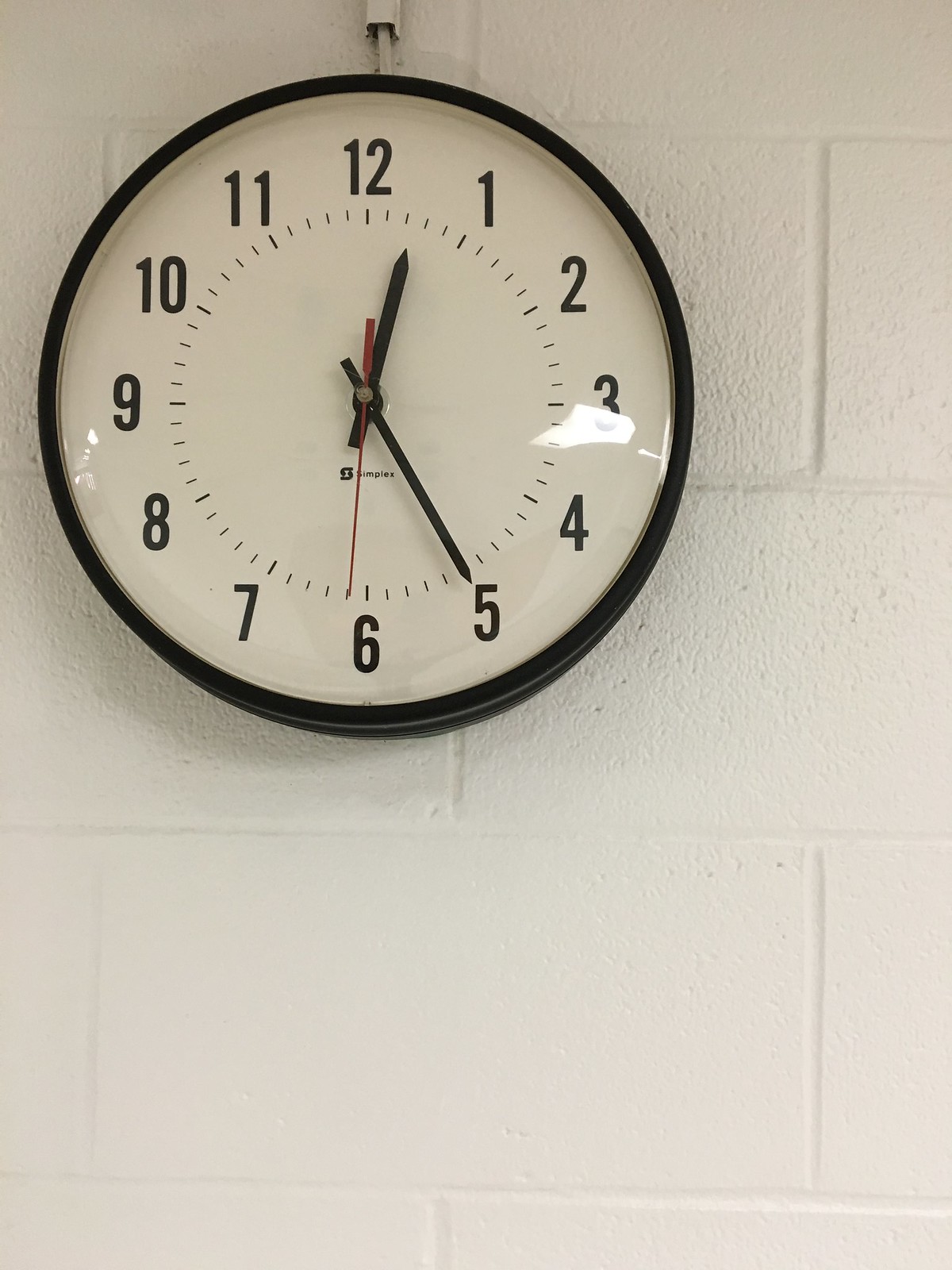This is an exceptionally clear photograph featuring a round clock mounted on a white brick wall. The clock is suspended by a white cord and secured with a white metal mount at the top. The clock face is a pristine, snow-white color, protected by a glass cover that subtly reflects light. The black numerals are bold and easily visible, complemented by black dash marks beneath them. The clock is equipped with two black hands and one striking red hand, allowing for precise time-telling. The clock casing is a sleek, rounded black, standing out against the crisp background. The high-quality image captures the delicate shadows cast by the clock on the textured white wall, highlighting the intricate lines and details of the bricks.